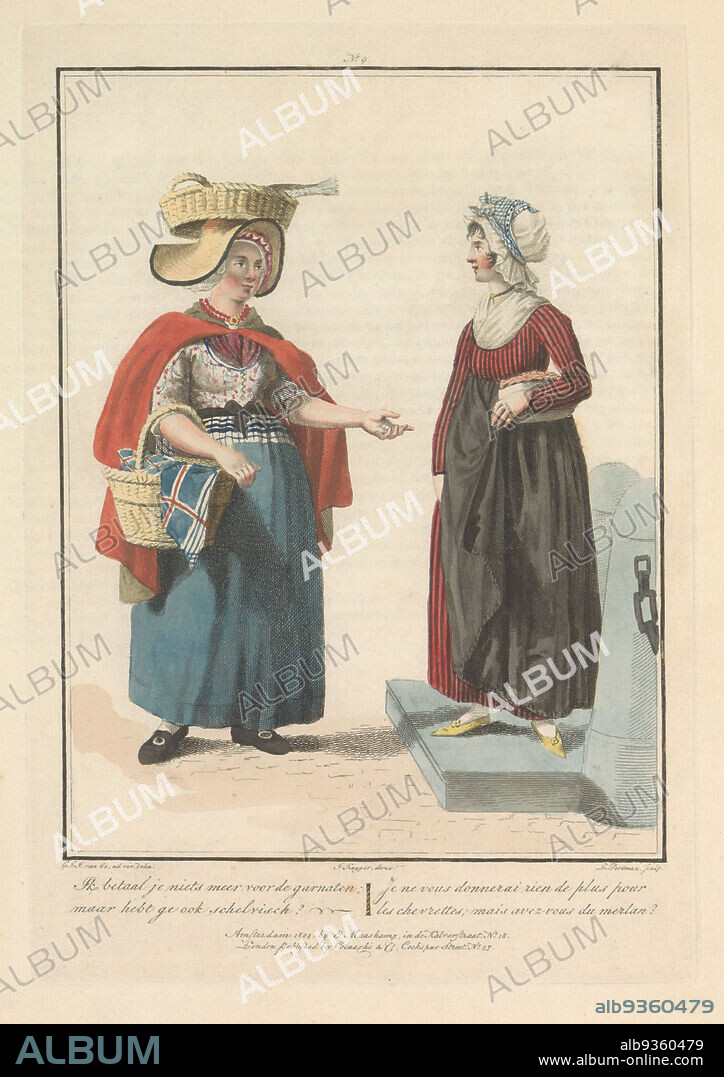The image is a highly detailed, vintage-style drawing or painting that appears to be a scanned page, heavily watermarked with the word "album" repeated diagonally across it. The scene features two women engaged in conversation, both dressed in medieval or old-fashioned attire. 

The woman on the left is characterized by her elaborate headgear, which includes a wide beach-like hat with a large wicker basket balanced on top. She wears a red cape over her shoulders, a long blue skirt, black shoes with white socks, and blue gloves. She carries another basket filled with materials that might resemble flags, including what some believe to resemble the Icelandic flag.

The woman on the right stands on a raised platform, reminiscent of a dock or port area, indicating a coastal setting. Her outfit consists of a red dress with black stripes, a large grey apron, and a white bonnet wrapped with blue material. She holds a substantial basket in her arms, which contains an indistinguishable object, possibly a pie.

The entire image is set against a tan background with a vertical black rectangular border. The bottom of the image displays an unreadable caption in a foreign language, along with the clear text "www.album-online.com," indicating its internet source.

The intricate detailing of their clothing and accessories, the period-specific attire, and the interaction between the figures make the drawing a captivating representation of a bygone era.